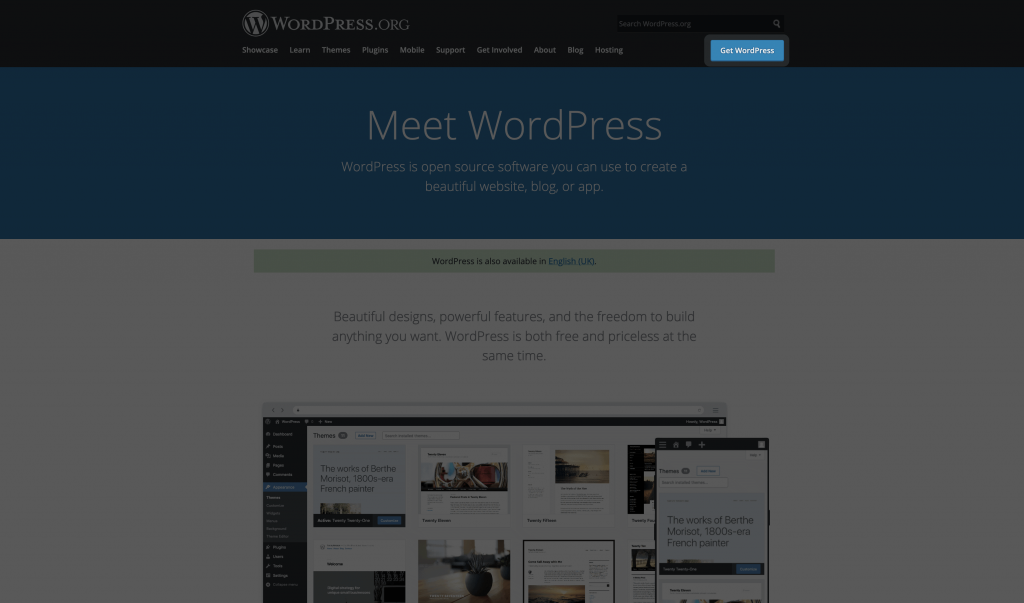The image depicts a WordPress promotional webpage. At the top, there's a black banner featuring the WordPress.org logo, which consists of a stylized "W" inside a circle, accompanied by white navigation text that reads: Showcase, Learn, Themes, Plugins, Mobile, Support, Get Involved, About, Blog, and Hosting. To the right, there's a blue rectangle button with white lettering that says "Get WordPress."

Below the banner, there's a blue section with white text that introduces WordPress, stating: "Meet WordPress. WordPress is OpenSource software you can use to create a beautiful website, blog, or app." The remainder of the page has a white background with a light green rectangle and dark text declaring, "WordPress is also available in English (UK)." 

Further down, there is more white text that emphasizes the platform's versatility: "Beautiful Designs, Powerful Features, and the Freedom to Build Anything You Want. WordPress is both free and priceless at the same time." 

Below this statement, a graphic illustrates a sample WordPress page, showcasing images and the word "Themes," suggesting it offers various theme options. On the left side of the graphic, there's a listing of different attributes one can select for their themes.